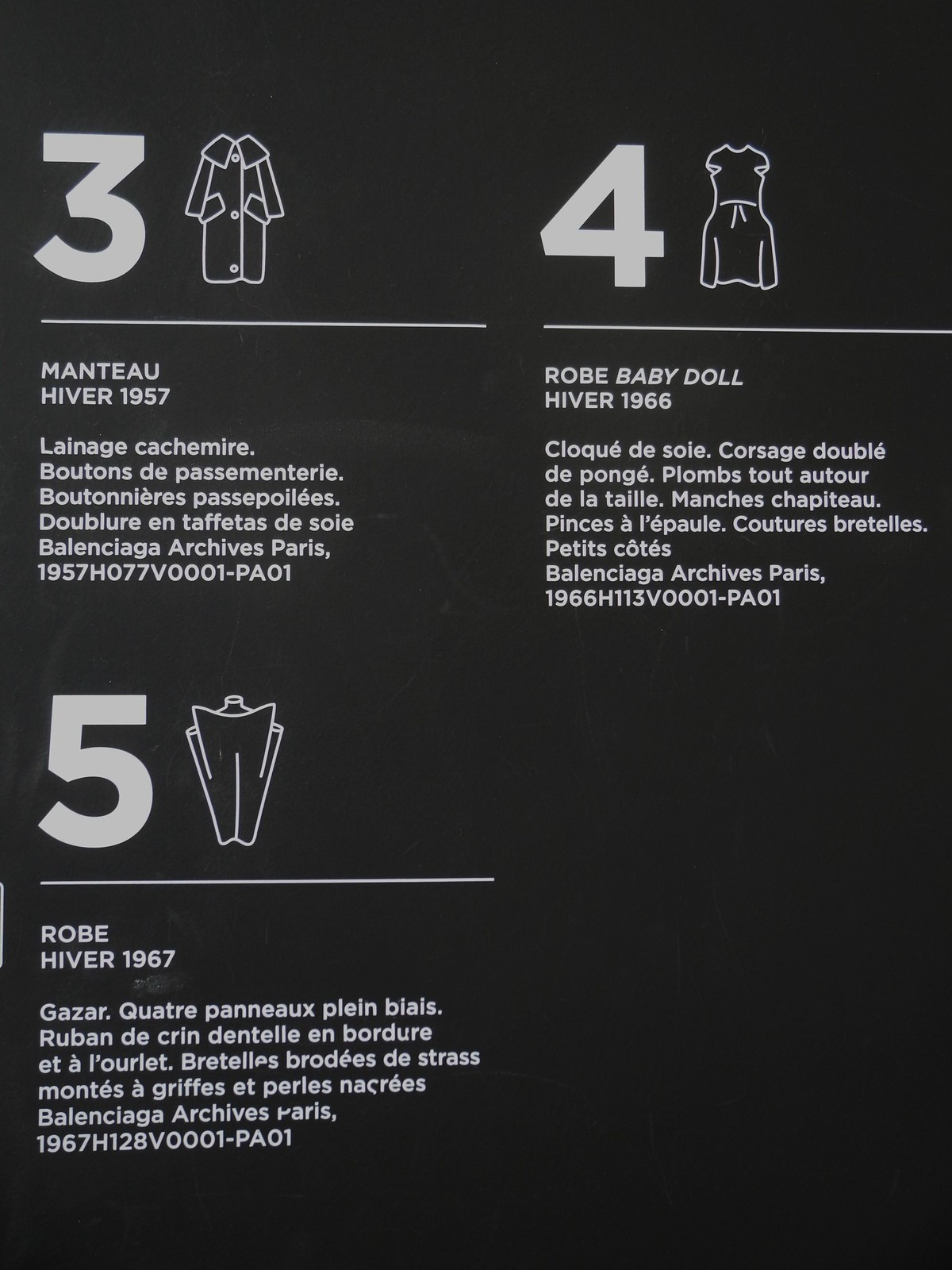The image depicts an informational placard with a black background and white font detailing notable clothing items from the Balenciaga Archives, primarily in French. The top left corner features the number three beside an illustration of a coat, titled "Mante Ohiva, 1957." In the top right corner, the number four is accompanied by a gown icon and the description "Robe Baby Doll Hiva, 1966." The bottom left corner shows the number five next to an illustration resembling an upside-down umbrella, labeled "Robe Hiva, 1967." Beneath these icons, additional texts in French detail the items further and include the notation "Balenciaga Archives Paris 1960 H113 V0001-PA01" or similar, respective to each piece. The placard likely serves as an exhibit card, showcasing these historical fashion pieces along with their associated years and archival references.